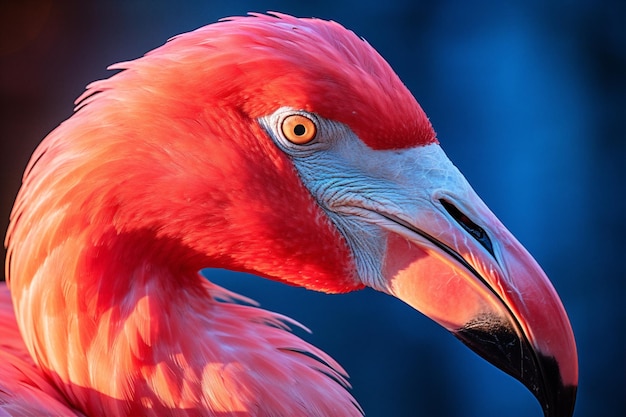This is a detailed close-up photograph of a flamingo's head, captured during sunset. The prominent features include the bird's pinkish skin, pink feathers, and striking orange eyes with a distinctive orangey-pink hue. The flamingo's large beak is predominantly pink with a black tip. The image showcases the flamingo in a side profile, with the backdrop consisting of a blurry blue and black gradient, which enhances the focus on the bird's vibrant colors and detail. The surrounding area around the eye is white, which contrasts with the rest of its pink plumage. The flamingo appears to be contemplative, perhaps searching for food, immersed in its thoughts, or simply observing its surroundings. The sunset adds a touch of warmth to the image, casting subtle shadows and a golden glow on the flamingo's head. The background remains out of focus, keeping the viewer’s attention firmly on the flamingo's detailed and vivid portrayal.